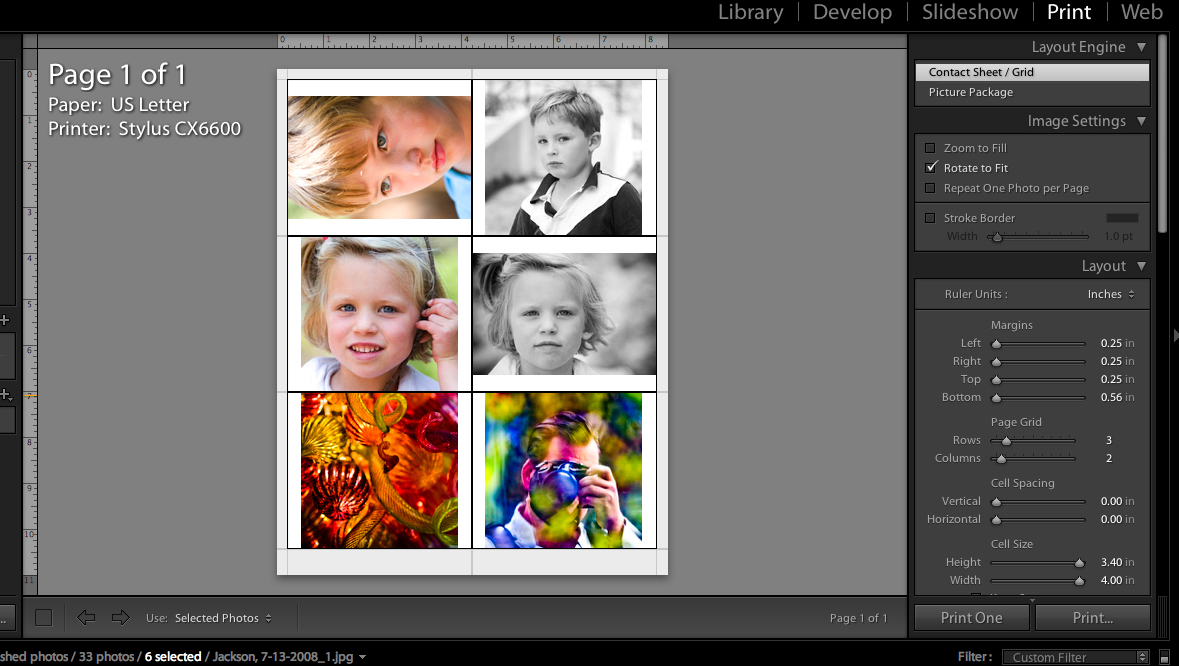The image is a screenshot from a computer displaying photo editing or printing software. The software interface has a gray background with a central area depicting a white page where a collage of six photos is arranged. The collage includes four images of children and two abstract or complex images. The top two photos feature a young boy; the left image in color shows him with white-blond hair and bangs, while the right image is a black-and-white portrait of him in a dark top with white trim. Below these, there are two images of a young girl, approximately four or five years old. The left image, in color, shows her with short light-colored hair and a hand up to her ear, while the right is a black-and-white portrait with a serious expression. The bottom left image is a jumble of red and yellow colors, possibly showing an open mouth with teeth, and the bottom right image, taken through colored filters, shows a man with short hair holding a camera to his eye, possibly a self-portrait.

The software interface also features a black border and various menus. In the top left, it states "page 1 of 1," "paper: US letter," and "printer: Stylus CX6600," indicating the paper size and printer model. On the right-hand side, there are layout and image settings, including options for size, margins, page grid, cell spacing, and print options. The upper right corner highlights the word "print," suggesting the user is preparing to print the page. At the bottom of the screen, some text indicates that there are 33 photos in total, with 6 selected for the collage. The file name is "Jackson 7-13-2008," possibly indicating a photo shoot from that date.